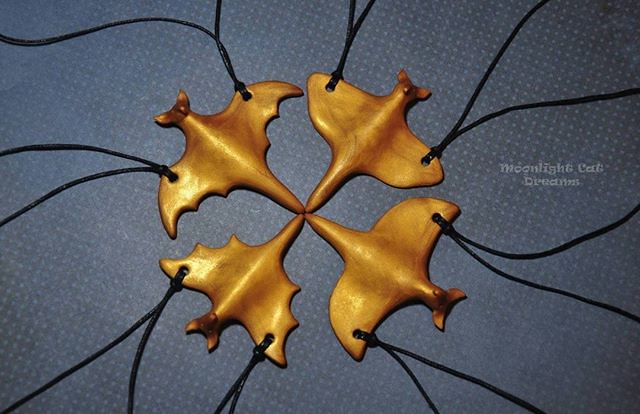The image features four identical bat-shaped figures, which appear to be either intricate gold figurines or delicate wood carvings. These bats have spread-out wings and look intended for decorative or hanging purposes, potentially even as a necklace. The bats are connected by black cords threaded through holes in their wings, forming a symmetrical arrangement. The left pair of bats show detailed, pointy wings, while the right pair have smoother wings. The entire setup is laid out on a hard, black surface adorned with white dots arranged in neat, smooth lines. A discreet watermark in the corner reads "Moonlight Cat Dreams."